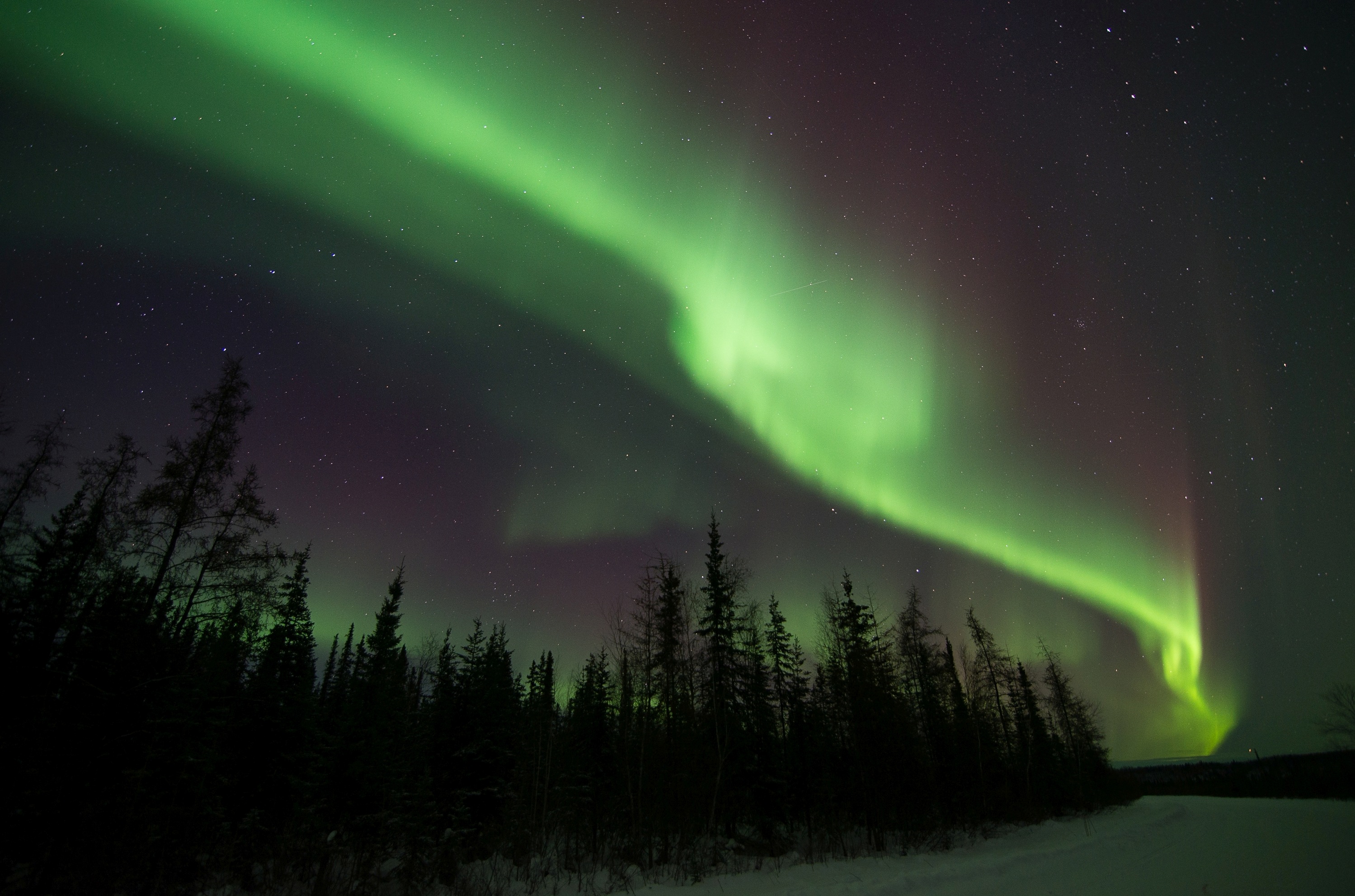A mesmerizing display of the northern lights dances across the night sky in this breathtaking nature photo. To the left, a dense cluster of dark pine trees stands tall, their silhouettes stark against the luminous backdrop. The sky is awash with mystical hues, as vibrant green bands of light cascade downward, intermingling with ethereal purple shadows. The aurora appears almost fluid, its movement creating a blurred, dome-like shape. This stunning spectacle arches gracefully towards the horizon, where shades of light and dark green merge seamlessly.

The ground below is blanketed in pristine snow, stretching out flat and unwavering, contributing to the scene's desolate yet serene atmosphere. The distant horizon fades into a black, clear sky, enhancing the contrast of the vivid aurora above. Scattered throughout the snow-covered landscape are clusters of resilient flowers, adding a touch of delicate beauty to the cold environment. In the far right corner of the image, the horizon is obscured by another layer of darkness, hinting at the presence of additional trees, hills, or a distant mountain range, completing this spellbinding portrayal of nature's grandeur.